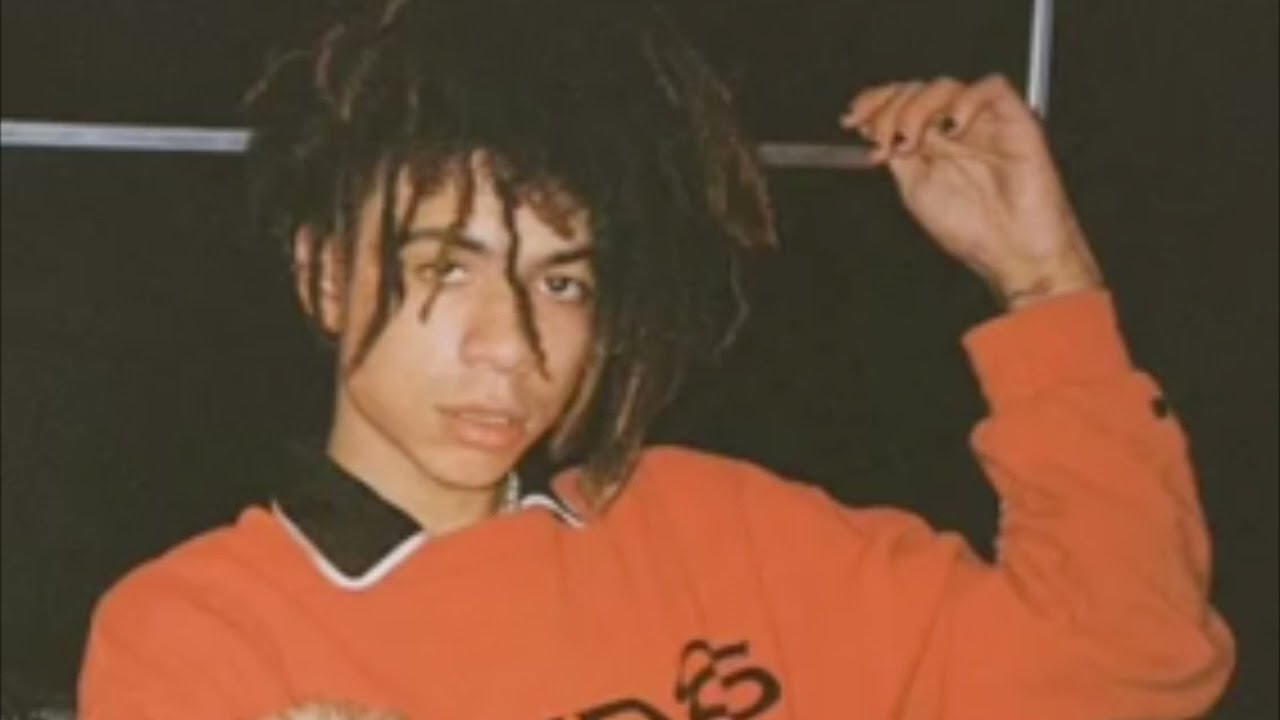The image appears to be an old photograph, likely from the late 80s to early 2000s, featuring a racially ambiguous young individual with light skin, possibly of mixed African-American descent. The person has dreadlocks that are piled on top of their head and swooped over to one side—longer on the right and shorter on the left. They are wearing an orange long-sleeve top with a black and white collar and some illegible black writing on the chest. The person is looking directly at the camera, and their left hand, adorned with black nail polish, is visible. The background is black, partially bordered by a visible silver frame at the top. The overall feel of the photograph evokes an old-school, film-developed aesthetic, possibly taken indoors.